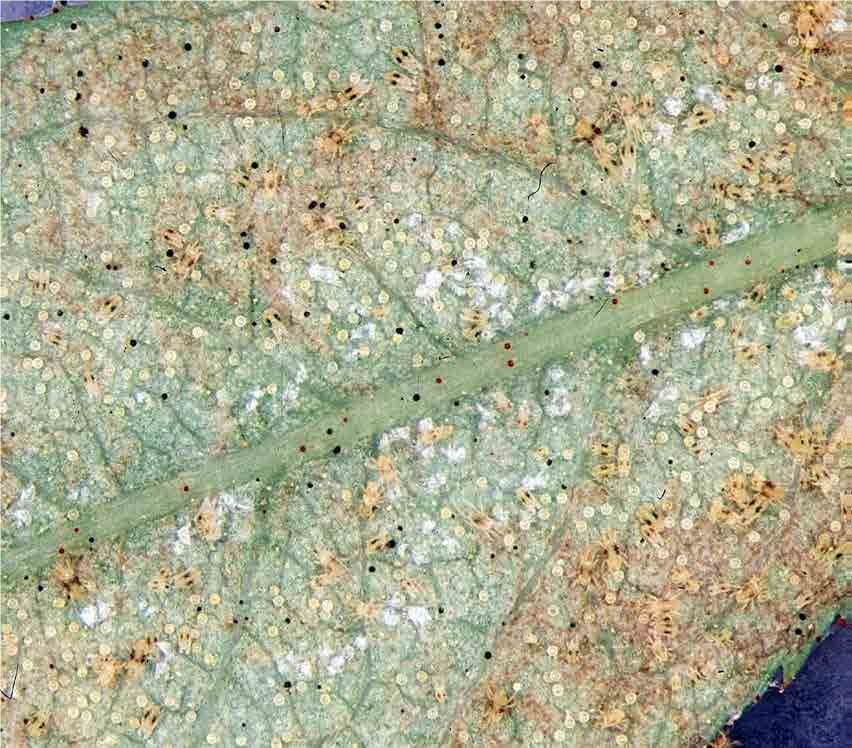The image appears to be an extremely close-up, macro shot of a leaf, possibly observed under a microscope, where the intricate details of the leaf's structure and surface anomalies are magnified. Dominating the composition is a pale green stem that traverses diagonally from the bottom left to the top right across the rectangular frame, slightly angled. Branching off from the central stem are green veins, creating a network that emphasizes the leaf's texture. The leaf, appearing light green, is covered in an assortment of speckles and patterns: white fuzzy-looking dots, yellow dots, and clusters of black and light brown specks. Additionally, patches of light brown and occasional dark blue on the edges are noticeable, contributing to its complex appearance. Some of these specs may represent parasitic organisms or cells dwelling on the leaf’s surface, highlighted by the pale tan parasites with black spots occupying parts of the leaf. These combined elements suggest the leaf is diseased or affected by some external factors, enhancing the detailed and almost surreal quality reminiscent of an art piece.